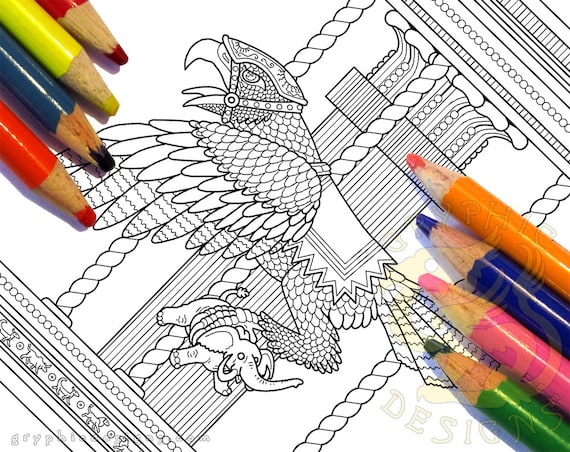This black and white illustration appears to be an intricate, adult coloring book page showcasing a fantastical scene. Central to the image is a gargantuan bird, possibly a medieval eagle, with detailed wings and armored features. Clutched in its talons is a small, sideways elephant, emphasizing the bird's enormous size. The background is dominated by a large, carousel-like structure with a cylindrical column at its center, supported by three intricately designed, spiral-shaped pillars that resemble barber poles, adding an optical illusion effect. The top and base of this structure are adorned with patterns of interlocking circles and squares.

In the upper left corner, four colored pencils, arranged in a descending order, with the colors dark red, yellow, blue, and orange, point downwards. Similarly, in the lower right corner, four more colored pencils, colored orange, purple, pink, and green, point upwards. The colors incorporated in the scene include black, white, orange, purple, pink, green, red, and blue, and yellow. Notably, a watermark or a graphic signature, "graphicdesigns.com," is imprinted in the lower-left area along with some translucent graphics reminiscent of gargoyles. The detailed and imaginative composition invites vibrant coloring to bring the fantastical carousel-like scene to life.